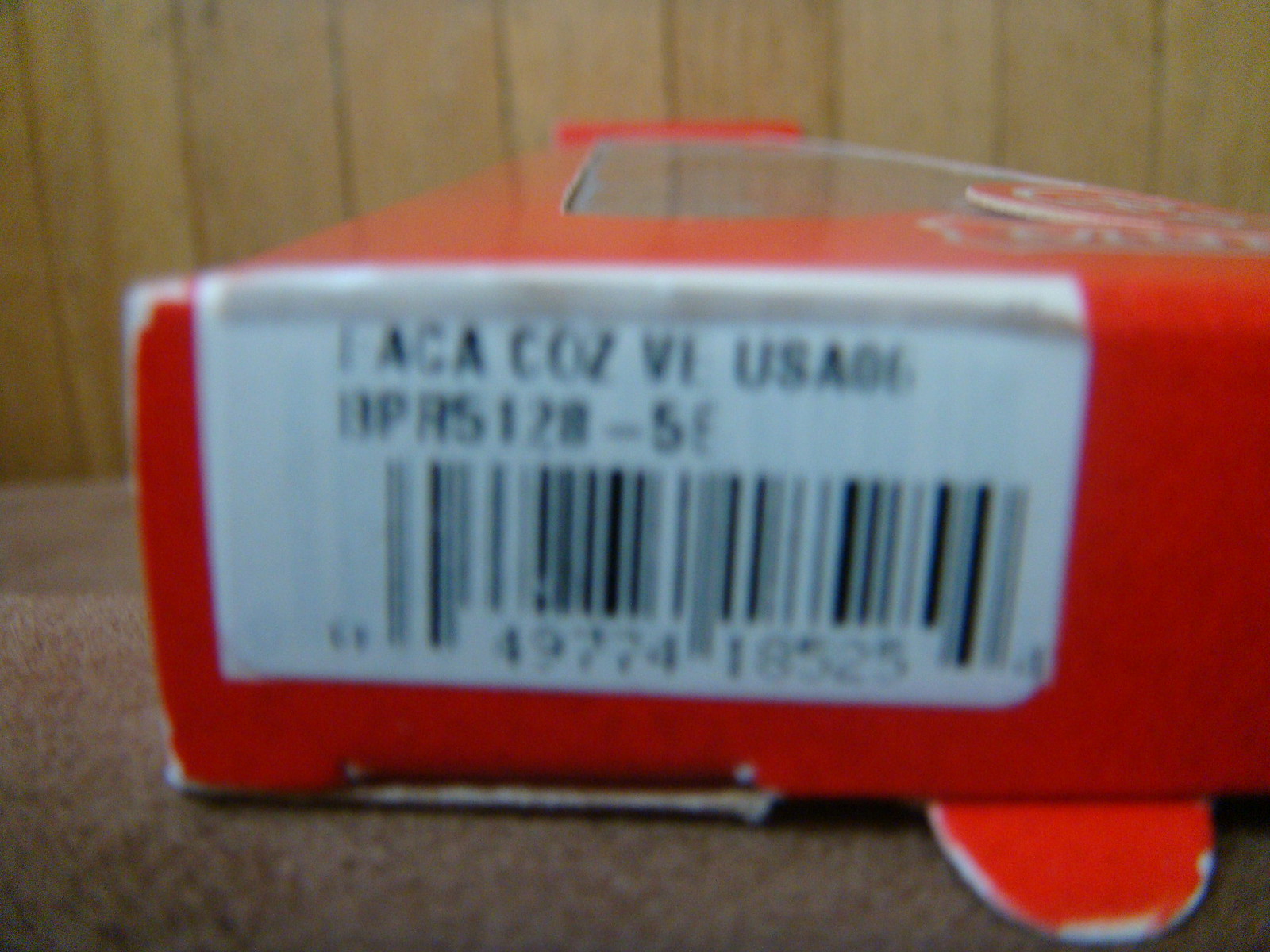A blurry and out-of-focus photograph features a white UPC code sticker affixed to an orangey-red cardboard box packaging. The package, resting on a beige low-pile carpet, has a clear plastic window on the top and noticeable foxing or wear around the edges. The barcode sticker, which is white with a black barcode across the bottom, seems to have text that reads "ACA COZ VE USAGE" followed by a product code that is hard to discern. The background includes a light-colored, vertically-planked wooden wall siding occupying the upper half of the image.